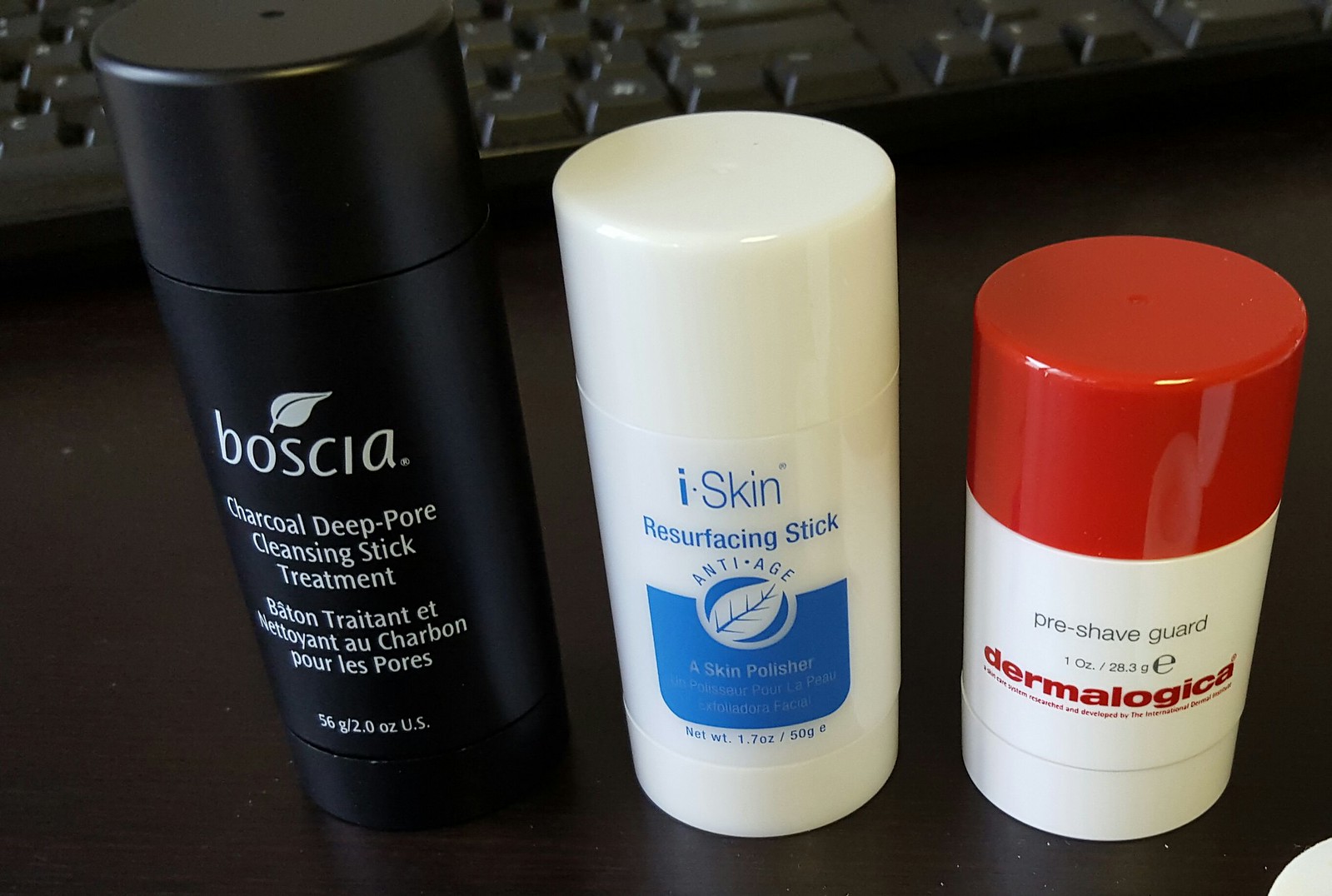A close-up photograph taken on a desk, likely near the person's computer setup as evidenced by the visible black keyboard in the background. The keyboard appears to have been pushed forward to make room for the three distinct cylindrical containers displayed in the foreground.

On the left is a black bottle labeled "Boscia Charcoal Deep-Pore Cleansing Stick Treatment," which is approximately the size of an average person's palm. The center item is a white plastic cylinder labeled "Eye Skin Resurfacing Stick Anti-Age," suggesting its use in anti-aging skincare routines. The third container on the right has a white body with a red lid and is labeled "Pre-Shave Guard," indicating its function as a pre-shave protective product. Both the black and white containers seem to be in stick form, similar to deodorant sticks, intended for targeted application.